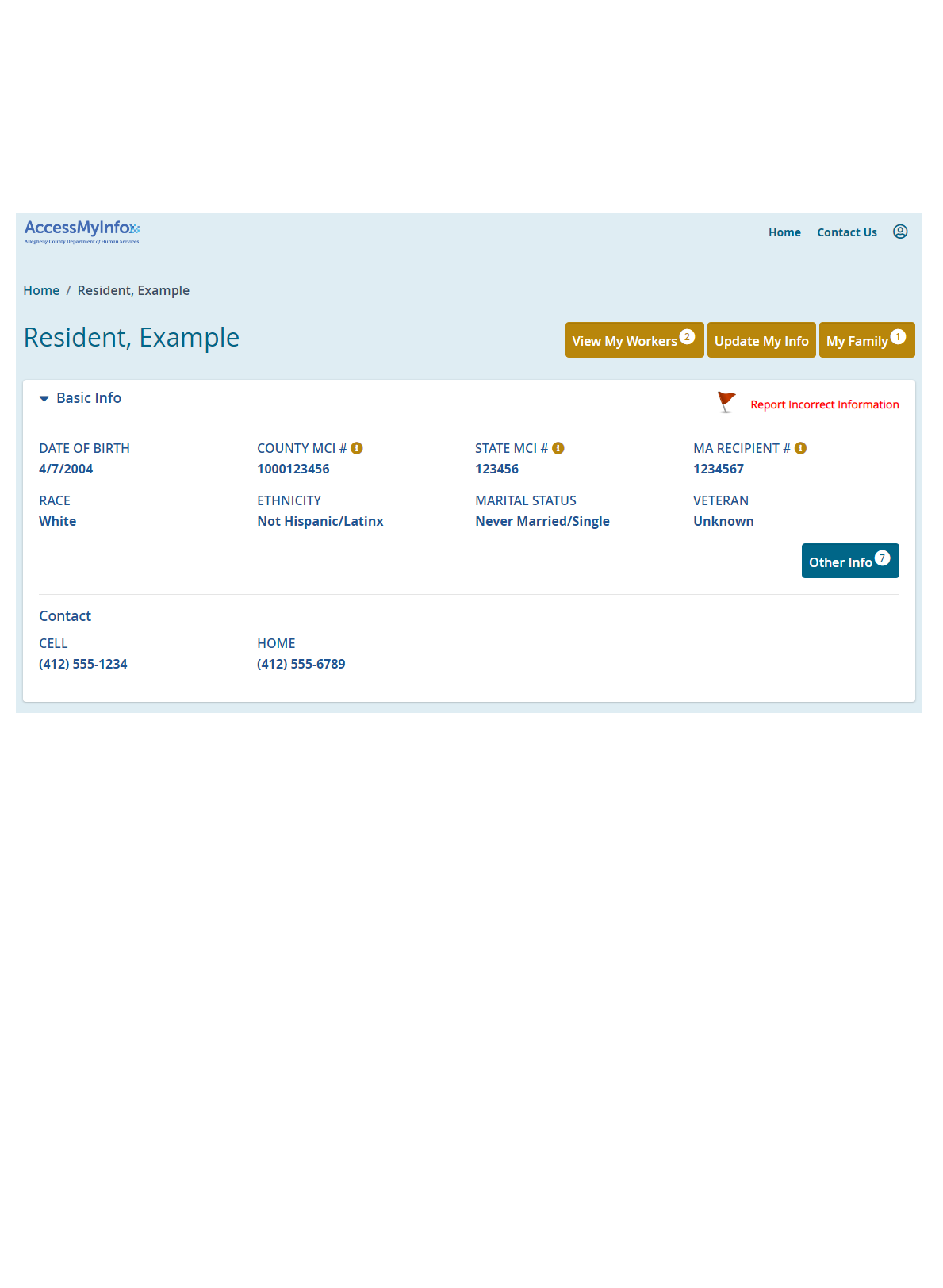This image depicts a computer screen showing an online interface labeled "Access My Info." The interface appears to be associated with Allegheny County, though the specific details are difficult to read due to the small print. Below the main heading, there is a breadcrumb trail reading "Home / Resident, Example," repeated twice in bold text.

To the right of the screen, there are several sections for managing personal and administrative details. One section titled "View My Workers" is marked with a notification badge displaying the number "2," indicating pending actions or updates. Another section, "Update My Info," is followed by "My Family," which has a similar notification badge with the number "1."

At the top right corner of the screen, navigation options include "Home" and "Contact Us," accompanied by a user profile icon.

Further down the page, personal information fields are displayed. The user’s date of birth is entered as "04/07/2004," and their race is listed as "White." Additional fields include contact details such as a cell phone number and a home phone number. Marital status is noted as "Never Married / Single." The form includes several other fields designated for personal information.